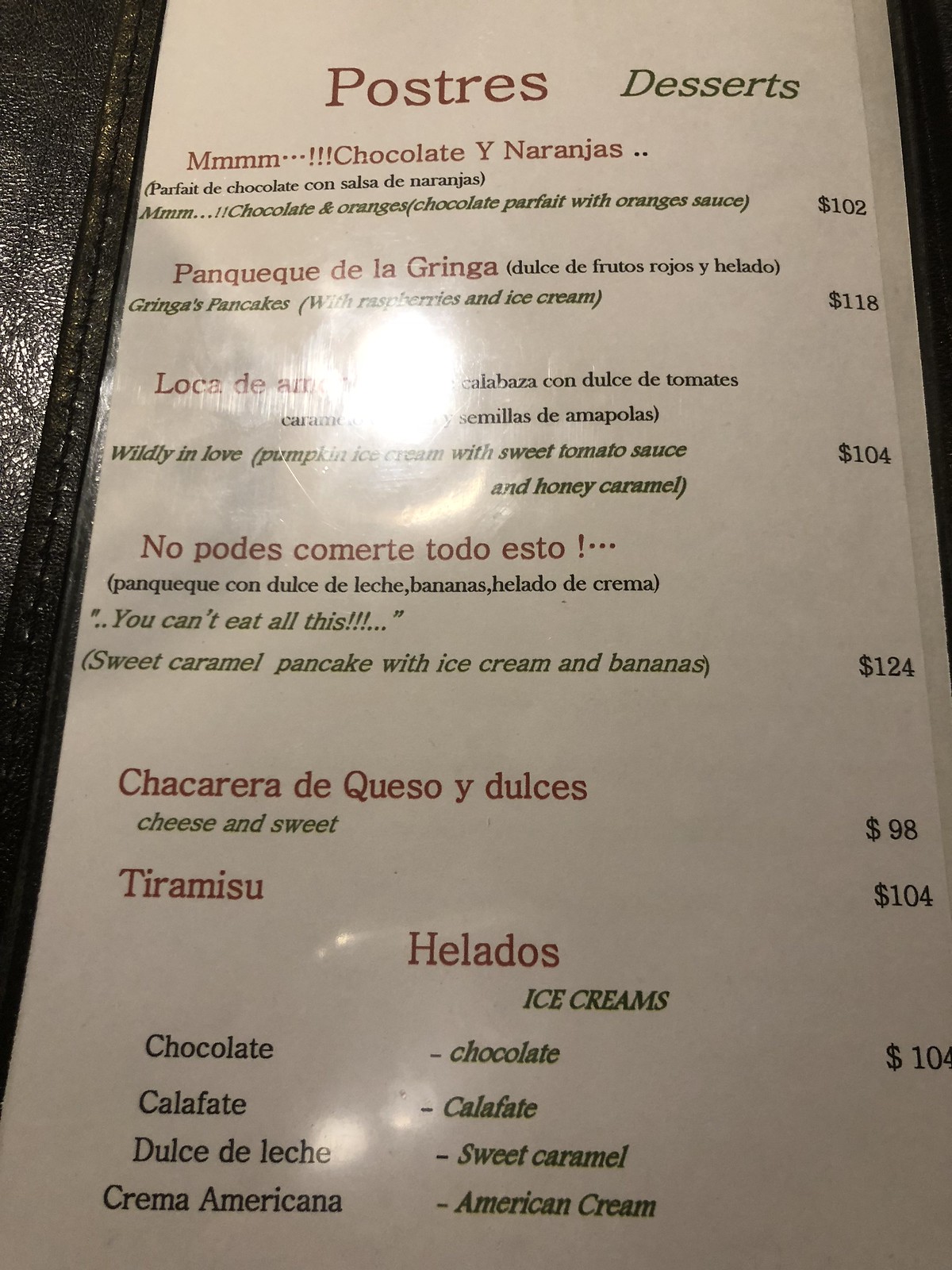The image displays a menu on a white background with a detailed list of desserts. At the very top, the menu features the title "Postres" followed by its English translation, "Desserts." 

The first item listed is "Mmm Chocolate," described in Spanish as "chocolate y naranjas." This dessert is a "Parfait de chocolate con salsa de naranja," which is translated into English as "Chocolate parfait with orange sauce," priced at 102. Presumably, this is in pesos, equivalent to approximately five dollars.

Next is "Panqueque de la Gringa," also labeled as "Gringa's pancakes" and "Dulce de frutos rojos y bebado." This section includes "You can't eat all this: Panqueque con dulce de leche, bananas, helado de crema," which means "Sweet caramel pancake with ice cream and bananas," priced at 124.

Following this, the menu lists "Chacarera de queso y dulces," translating to "Cheese and sweet," priced at 98. There's also "Tiramisu," priced at 104, and a section for "Helados" (Ice Cream).

This menu offers a tantalizing variety of desserts with both Spanish and English descriptions, making it accessible to a broader audience.